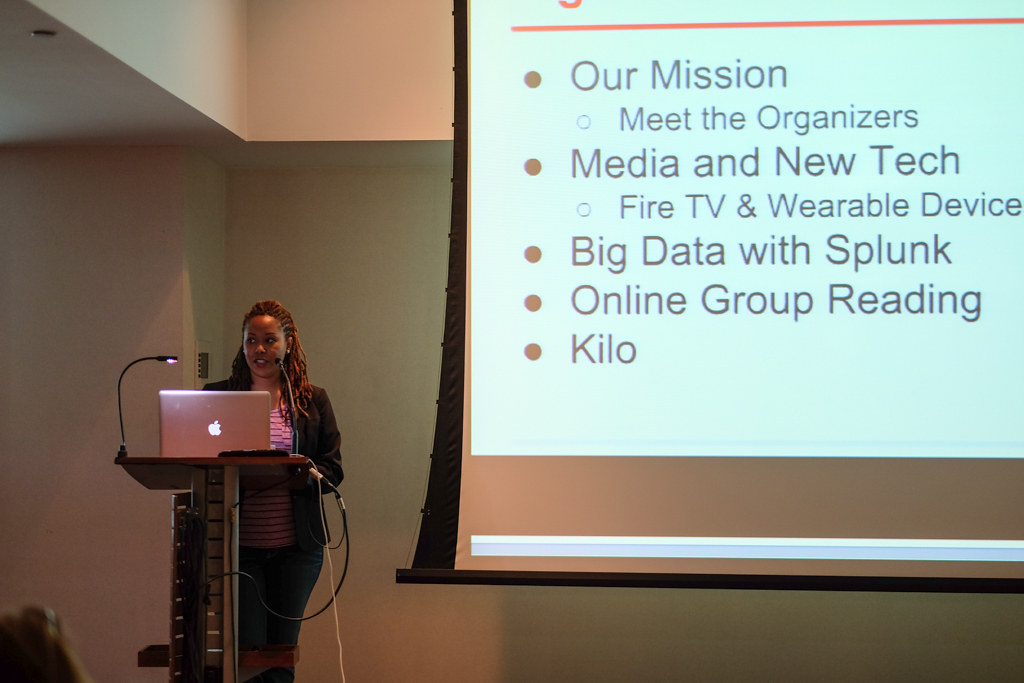The image captures an African-American woman standing at a podium, engaged in giving a presentation in what appears to be a classroom or small event setting. The room is dimly lit, with more light coming from an open area in the ceiling. She is positioned on the lower left side of the picture, using an Apple laptop with two microphones in front of her—one close to her mouth and the other off to the left side. Several wires run across the podium. Dominating the right side of the image is a large projection screen displaying a slide with a white background, organized into bullet points. The text on the slide reads: “Our Mission, Meet the Organizers, Media and New Tech, Fire TV and Wearable Devices, Big Data with Splunk, Online Group Reading, Kilo.” The colors in the scene include hues of very light bluish-green, brown, reddish, beige, black, grays, and whites, giving the setting a balanced, albeit subdued palette. This scene likely depicts a school event or an organized speaking event focused on technological and organizational themes.